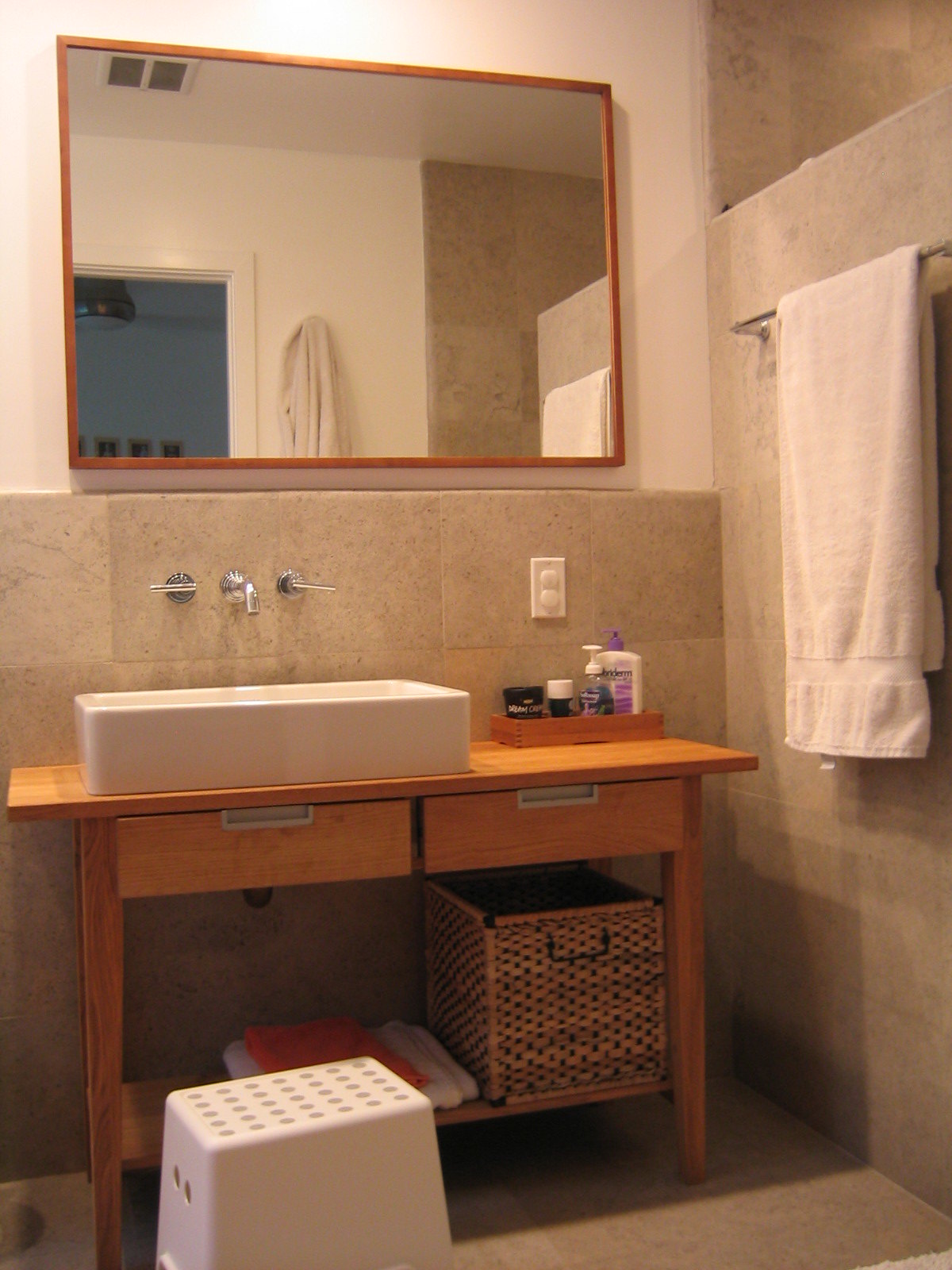This nighttime photograph captures a meticulously organized bathroom. Illuminated by an overhead lamp, the scene focuses on a rectangular white basin perched on a wooden counter. The counter features two drawers and a shelf below, which houses a wicker basket on one side and neatly stacked towels on the other. 

Above the basin, large pale gray tiles extend halfway up the wall, transitioning to a fully tiled wall in the shower area visible in the mirror's reflection. The sink is equipped with a sleek mixer tap emerging from the tiled wall. A white plastic step stool, designed for children with lift holes on each side and perforations on the top, sits next to the counter.

On the right side of the basin, a wooden box holds various toiletries such as hand soap and moisturizer, strategically placed below two plug points for charging electric devices like toothbrushes or shavers. Enhancing functionality, a stainless steel towel rack is mounted higher on the right wall, displaying a neatly hung white towel.

A large mirror with a wooden frame hangs above the basin, reflecting the tiled shower area ceiling and a robe or towel hanging from a hook. The floor is adorned with matching large gray tiles, creating a cohesive and elegant look throughout the space. The reflection of the darkened doorway in the mirror, combined with the ambient lighting, suggests the photograph was captured at night.